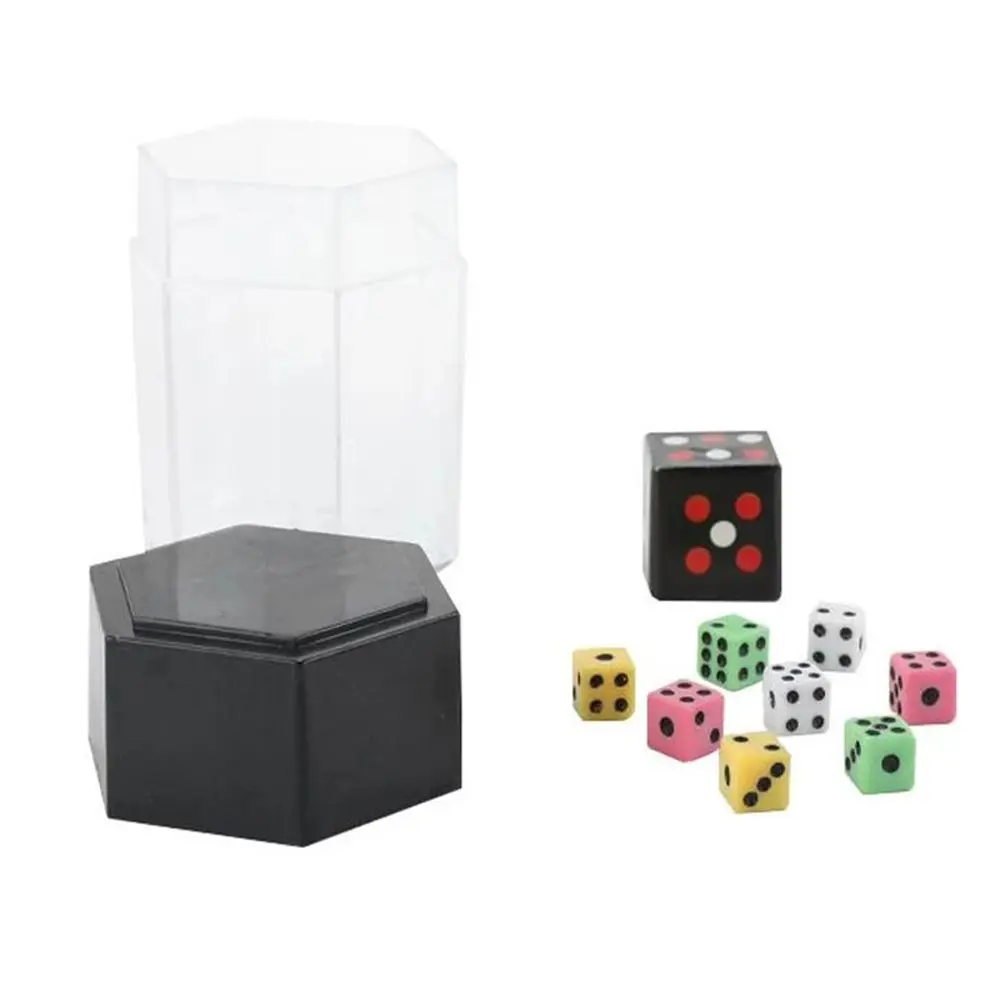This image depicts a set of dice designed for tabletop games, such as Dungeons and Dragons. The dice set is displayed on a white background, suggesting a product photo likely intended for a retailer's website. To the left of the photo is an octagonal case consisting of a black, octagon-shaped base and a semi-transparent plastic topper, which serves both as storage and potentially a rolling surface to keep the dice contained. 

The dice themselves are a vibrant array of small pieces in colors such as yellow, pink, green, and white, each showing different numbers. Notably, there is one large black die among them, distinctively marked with red and white dots, with the number five represented by four red dots and one white dot. This larger die contrasts with the smaller, multi-colored ones, adding a focal point to the image. The case and its components appear designed to carefully store and perhaps display these dice, enhancing their appeal for hobbyists and role-playing enthusiasts.